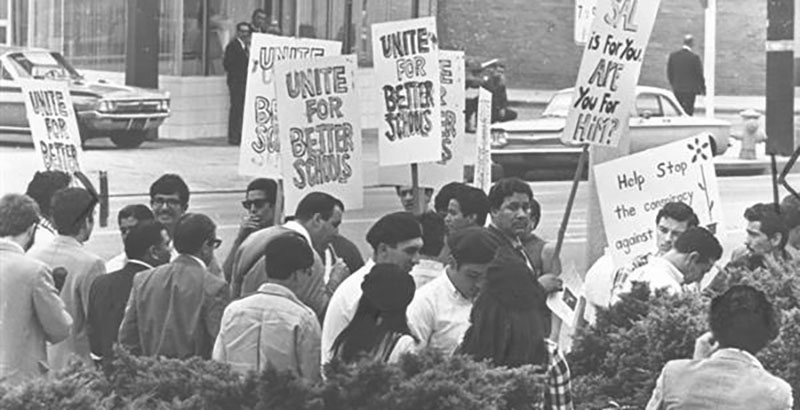This black-and-white photo, likely from the 1980s, captures a group of about 15 to 20 protesters, consisting mostly of men with a few women with long hair. They are standing serious-faced, holding various protest signs. Some signs read "UNITE FOR BETTER SCHOOLS" and "HELP STOP THE CONSPIRACY AGAINST..." with part of the text obscured by someone's head. One sign also includes a diagram of a flower. The protesters, some wearing glasses, appear to be either teachers or union members advocating for improved schools. They are gathered on a sidewalk bordered by bushes near a street with old-school cars parked in the background. The image offers a rear view of many of the individuals, emphasizing the collective action of the group.